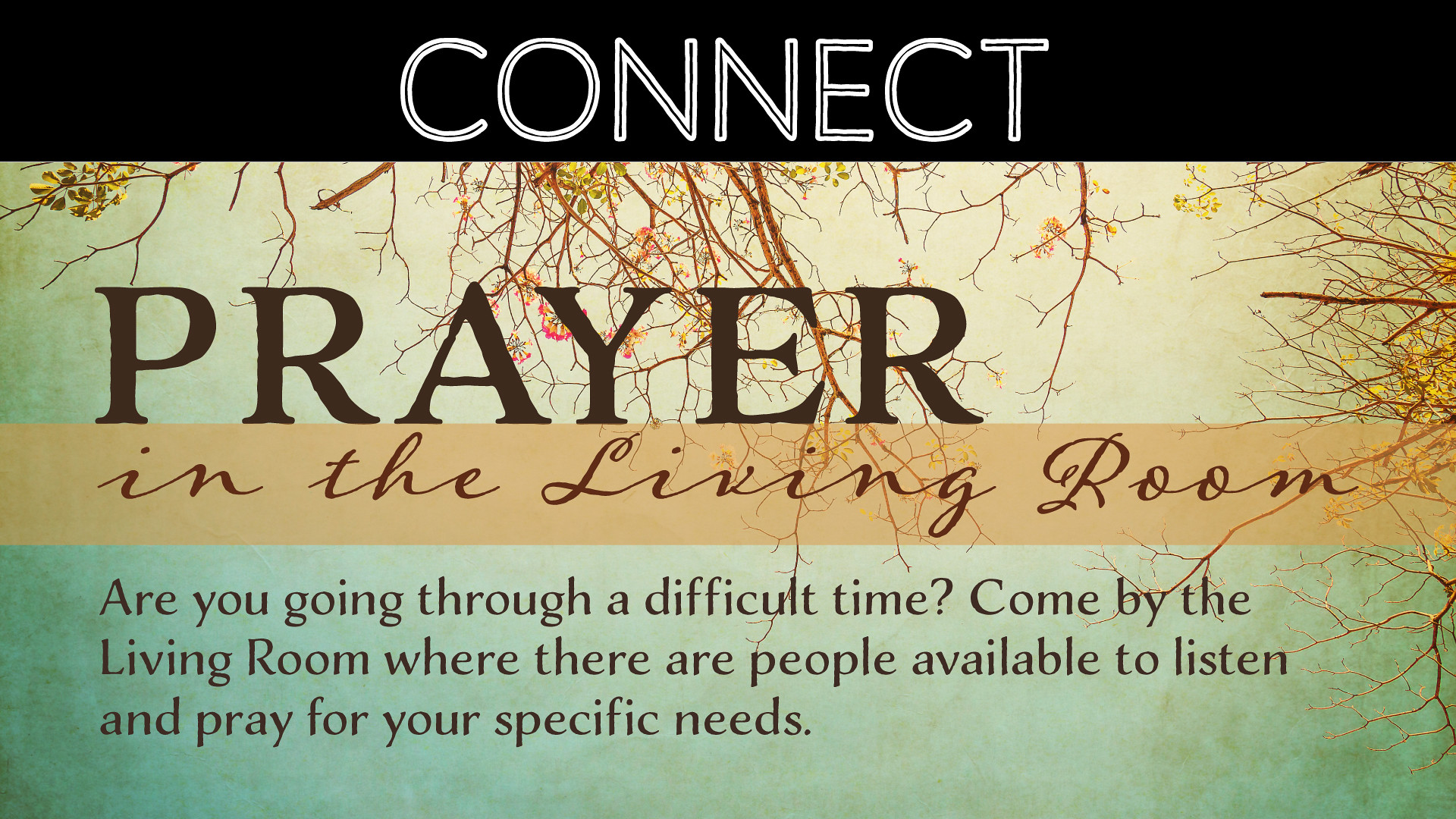This full-color promotional flyer features four distinct panels. The top panel is black with bold white text that reads "CONNECT." The second panel presents an upward view from the ground, showcasing mostly bare tree branches with a few leaves, set against a sky backdrop. In large black text, it simply says "PRAYER." Below this, a thin brown border contains the words "IN THE LIVING ROOM" in brown cursive text. The bottom panel, primarily blue with a greenish hue, contains more tree branches and some pink flowers. It asks, "ARE YOU GOING THROUGH A DIFFICULT TIME?" followed by an invitation: "Come by the living room, where there are people available to listen and pray for your specific needs."